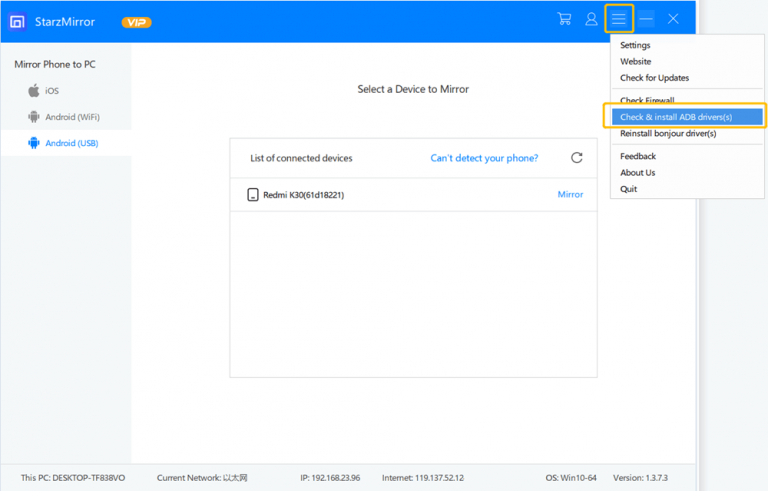The image depicts a user interface for an application or software named STARSMIRRORVP, designed for mirroring phone screens to a PC. 

In the header, which is styled with a blue background, the software's name "STARSMIRRORVP" is prominently displayed. To the left of this, the interface provides essential information about its functionalities, such as the ability to mirror phones to PCs from iOS and Android devices via Wi-Fi and Android USB.

Below this header, the main body of the interface features a central white rectangle. At the top of this section, there is a prompt stating "Select a Device to Mirror". Underneath, there are options and instructions: "List of Connected Devices," a troubleshooting link labeled "Can't Detect Your Phone," and a "Refresh Button." Also, an identified device "Redmi K30" with the ID "(6 1 D 1 8 2 2 1)" is listed, beside which there is a blue button labeled "Mirror."

On the right side of the interface, a vertical menu displayed in a white box offers several choices. The options are listed in black text as follows: "Settings," "Website," "Check for Updates," and "Check Firewall." Below these, a blue rectangle with an orange outline contains the text "Check and Install ADB Drivers." The menu continues with more options: "Reinstall Bonjour Drivers," "Feedback," "About Us," and "Quit."

At the bottom of the image, there is a courteous sign-off: "Thank you for watching!"